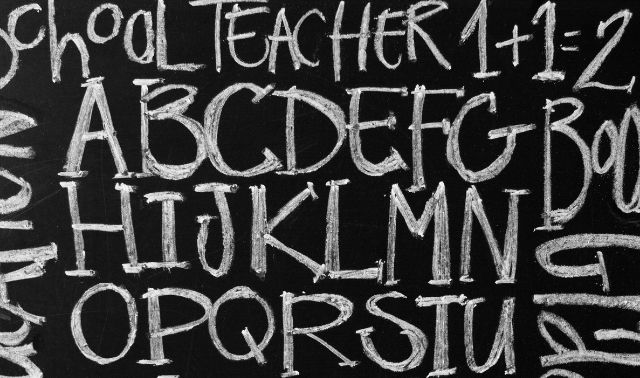The image presents a black, rectangular chalkboard, adorned with various writings in white chalk. At the center, the alphabet is written in a sequence from A to U, arranged in a square pattern. Surrounding this central block, additional text is scattered and angled, including phrases such as "school teacher" and the equation "1 + 1 = 2." On the far left, the word "school" is partially visible, starting with an "S" but the rest of the word is cut off, displaying just "C-H-O-O-L." On the extreme right, an indecipherable word appears, possibly beginning with "B-O-O-G" followed by indistinct letters. The overall layout is clean, suggesting the use of a small, well-maintained chalkboard, with all elements drawn carefully in white chalk.